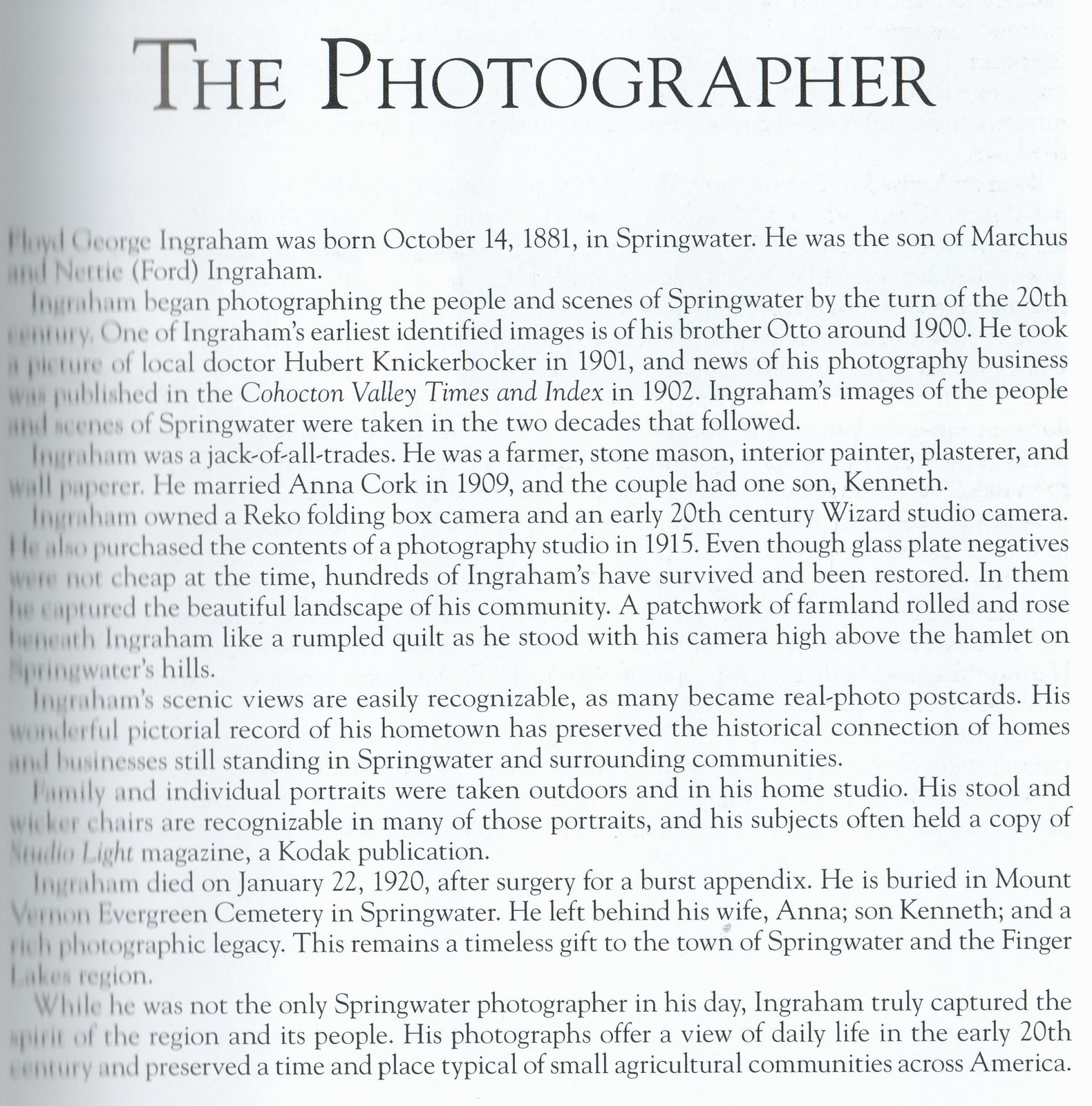The image is a black and white tribute piece or obituary on a single sheet of paper, dedicated to Floyd George Ingram. At the top, in large letters, it identifies him as a photographer. Below that, it notes that Ingram was born on October 14, 1881, in Springwater, as the son of Marcus and Nettie Ford Ingram. The text continues in several paragraphs, detailing his life and work. Ingram began photographing the people and scenes of Springwater by the turn of the 20th century, capturing significant local figures such as his brother Otto around 1900 and Dr. Hubert Knickerbocker in 1901. His burgeoning career was announced in the Cohoctin Valley Times and Index in 1902. Over two decades, he documented the daily life of Springwater’s agricultural community. Known as a jack-of-all-trades, Ingram also worked as a farmer, stone mason, interior painter, plasterer, and wallpaperer. He married Anna Cork in 1909, and they had a son named Kenneth. Ingram owned several cameras, including a Ricoh folding box camera and a wizard studio camera, which he acquired along with the contents of a photography studio in 1915. The tribute concludes by acknowledging that while Ingram was not the only photographer in Springwater during his time, his photographs uniquely captured the spirit of the region and its people, preserving a glimpse of early 20th-century life typical of small American agricultural communities.